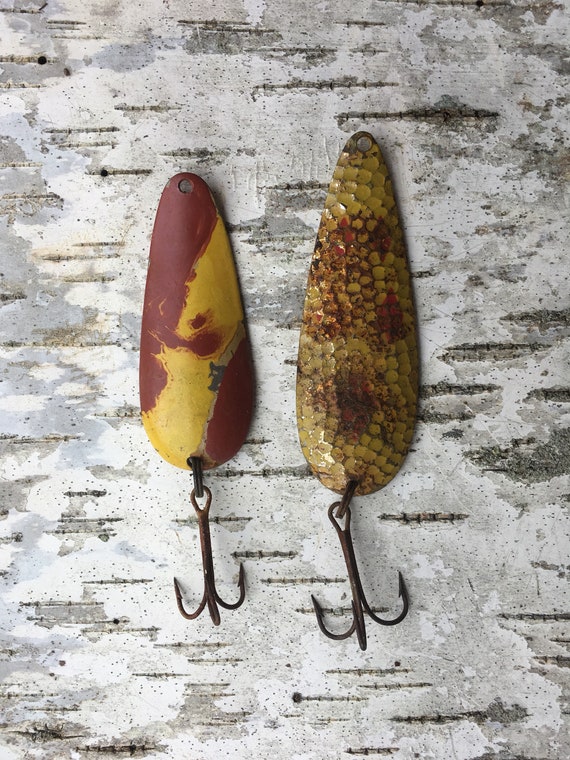The image showcases two vintage fishing lures, likely made of ceramic or metal, placed centrally on a distressed, grey surface resembling paper birch bark with white and dark line accents. Both lures are elliptical in shape with black metal hooks attached at the bottom, each featuring four prongs for fishing. The smaller lure on the left is painted in a maroon or dark pink and pale yellow color scheme, indicating age and wear. The larger lure on the right has a textured top with speckled yellow bits and a base of yellow and brown hues. The overall setting and style emphasize a classic fishing theme.